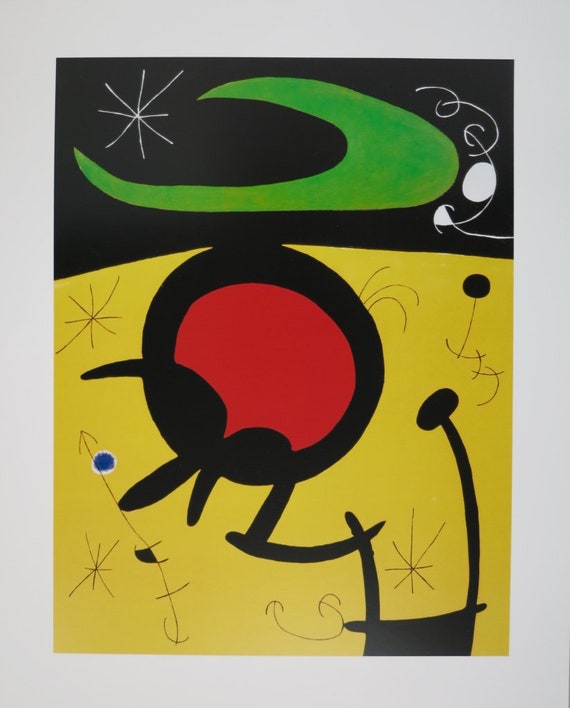This is a detailed drawing featuring a vibrant and surreal night scene. The background consists of a black sky occupying the top quarter of the image, transitioning into a yellow landscape that covers the bottom three-fourths. Dominating the upper section is a crescent-shaped green moon with its curved side facing right. To the left of this moon is a depiction of a star, represented by intersecting lines rather than a traditional star shape. On the right side of the moon, there are some white, curved, squiggly lines. Below this celestial scene, within the yellow ground, lies a central figure—a ladybug. This ladybug is meticulously drawn with a bold black outline encircling its red body, featuring two black eyes and two black antennas, the left one being slightly longer with a knob at the end. The design of the ladybug and the overarching whimsical elements create a captivating contrast against the stark night sky.